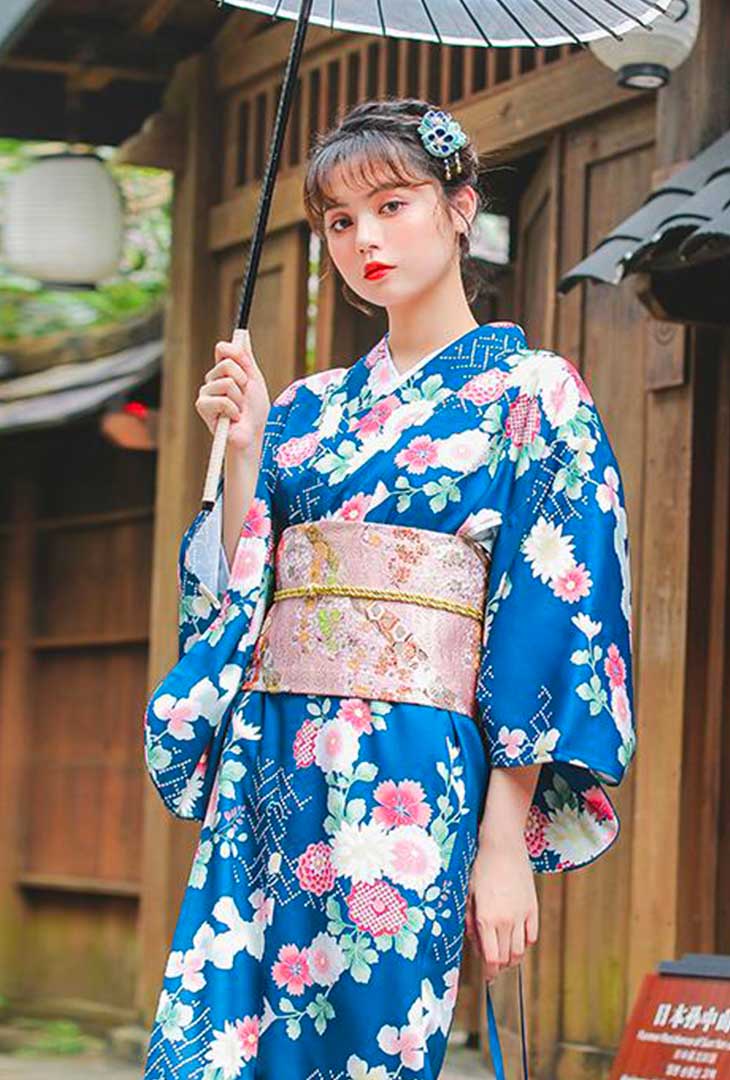This close-up, portrait-oriented photograph captures a young woman dressed in traditional Japanese attire. She wears a royal blue silk gown adorned with white and pink flowers, green leaves, and subtle white geometric designs. Cinched at her waist is a large, wide pink obi belt decorated with flower appliques and secured with a gold rope.

Her short, dark hair is pulled back, with gently resting bangs framing her face, accented by a blue and turquoise beaded hairpiece. The woman holds a traditional Japanese parasol with a black handle and a white underside featuring black spokes above her head in her right hand. In her left hand, she carries a bag with blue straps. 

She stands before a traditional Japanese wooden building, characterized by brown roof tiles and white lanterns hanging from the eaves, creating a serene backdrop. Her pose is slightly tilted to the right, with a subtle, emotionless expression, emphasizing the serene and dignified nature of her presence.